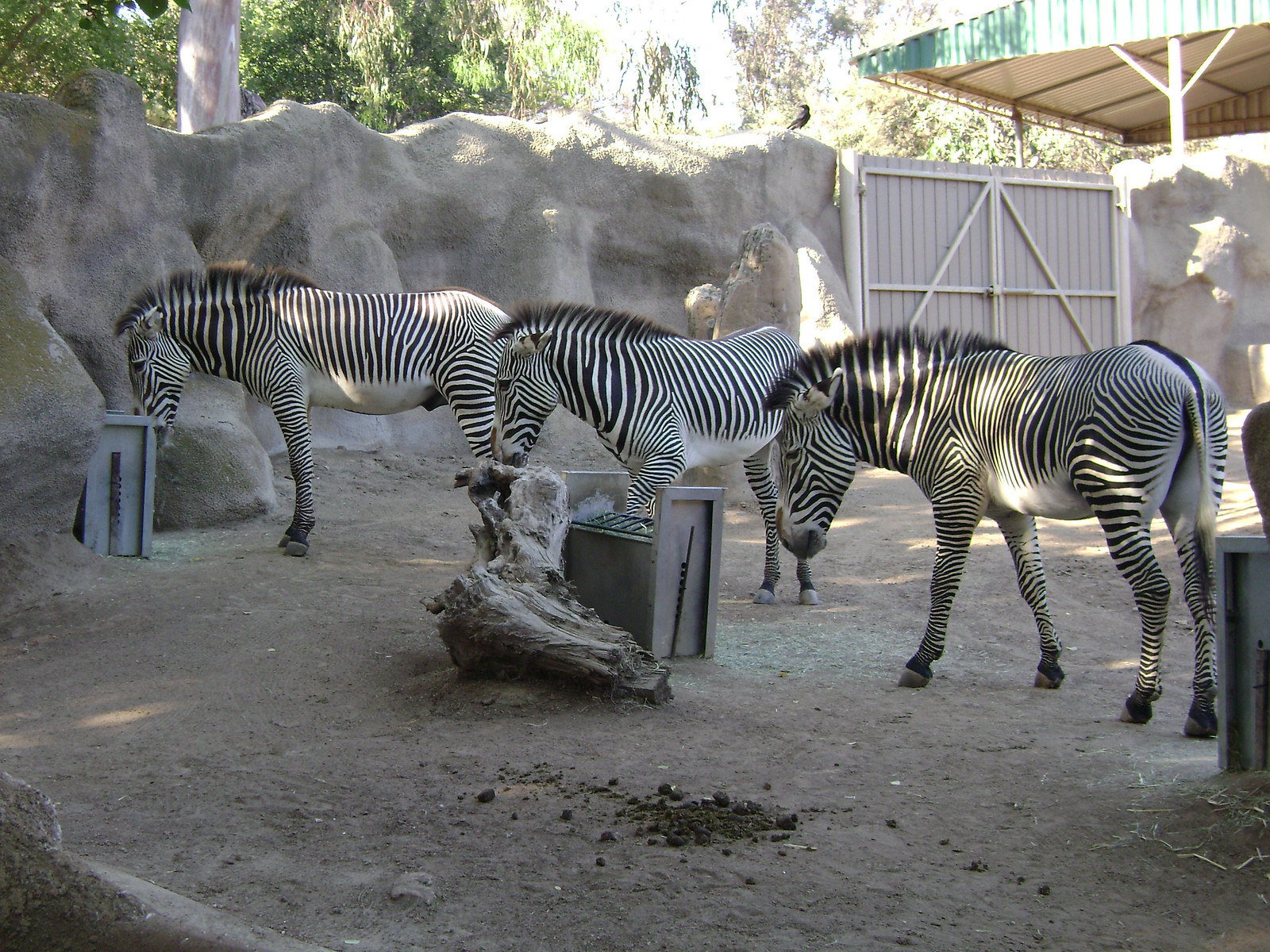The image captures a daytime scene of three zebras in a zoo enclosure, featuring their characteristic black and white striped bodies, short manes that stick straight up, dark eyes, and dark muzzles. All three zebras are positioned as if they're eating or drinking from three box-like feeders that are gray and light blue in color, lined up in the middle of their sandy, gravelly habitat. The enclosure itself is bordered by tall, stone or artificial stone walls, with a large solid wooden gate prominently in the center. In the upper right-hand corner, there is a green tin shade structure casting shadows throughout the area. The backdrop features tree trunks and deciduous vegetation, indicating a sunny day with light streaming through and creating various shadows on the enclosure’s elements. Scattered around the ground are darker rocks or perhaps defecation, adding texture to the dusty floor. Additionally, there's a small log lying on the ground, hinting at elements of enrichment within the enclosure.